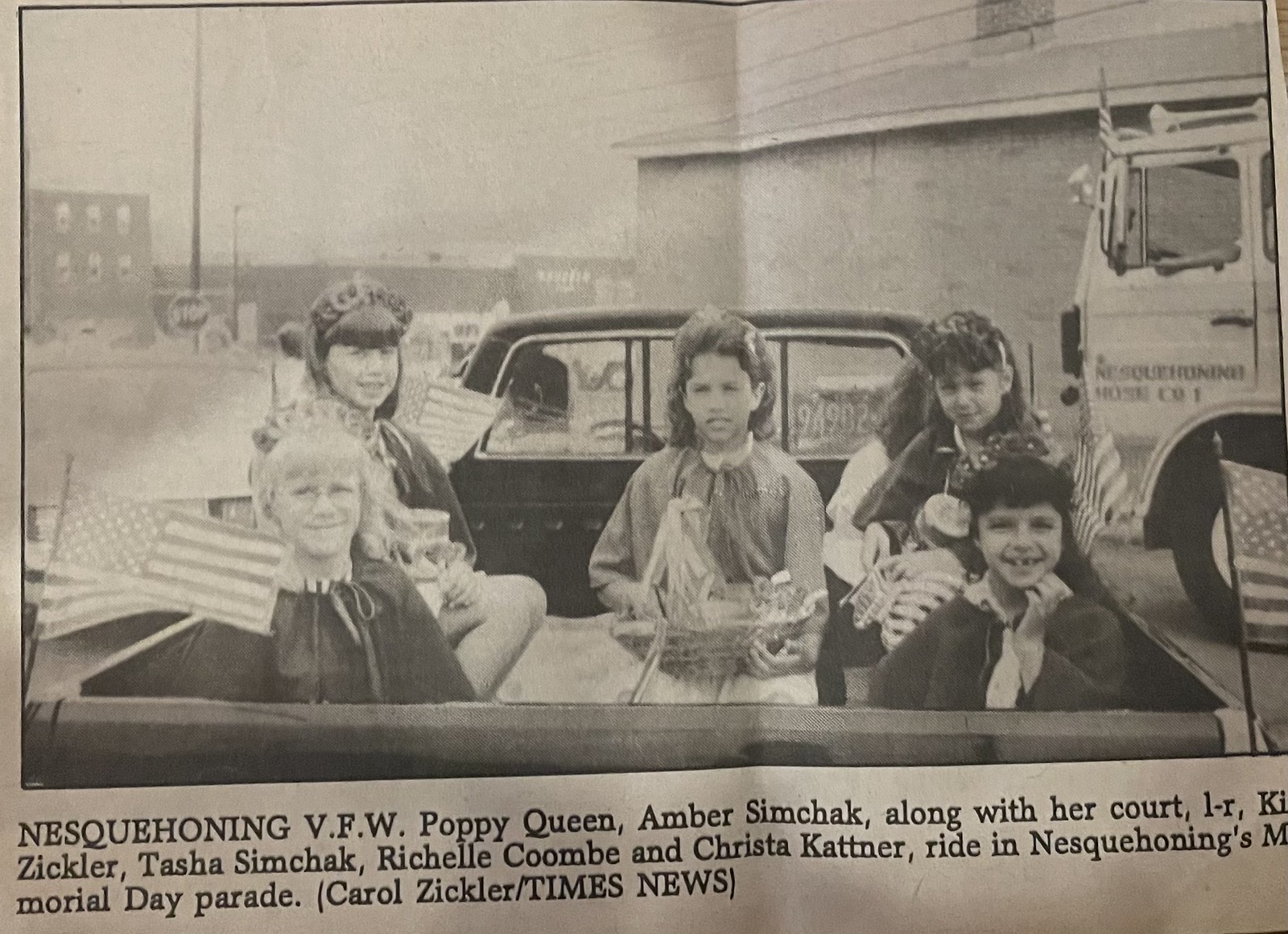The black-and-white photograph, resembling a vintage newspaper clipping, captures a moment from Nesquihoning’s Memorial Day Parade. The image features five girls sitting in the back of a pickup truck, all looking towards the camera with smiles. The truck is adorned with four American flags positioned in each corner of the truck bed. The girls are identified in the caption as Nesquihoning VFW Poppy Queen Amber Simchak and her court members: Zickler, Tasha Simchak, Rochelle Kuhm, and Krista Kattner. The scene includes a partially visible white truck cab and a large cement building in the background. The photo credit is given to Carol Zickler of the Times-News, hinting that she might be the mother of one of the court members.